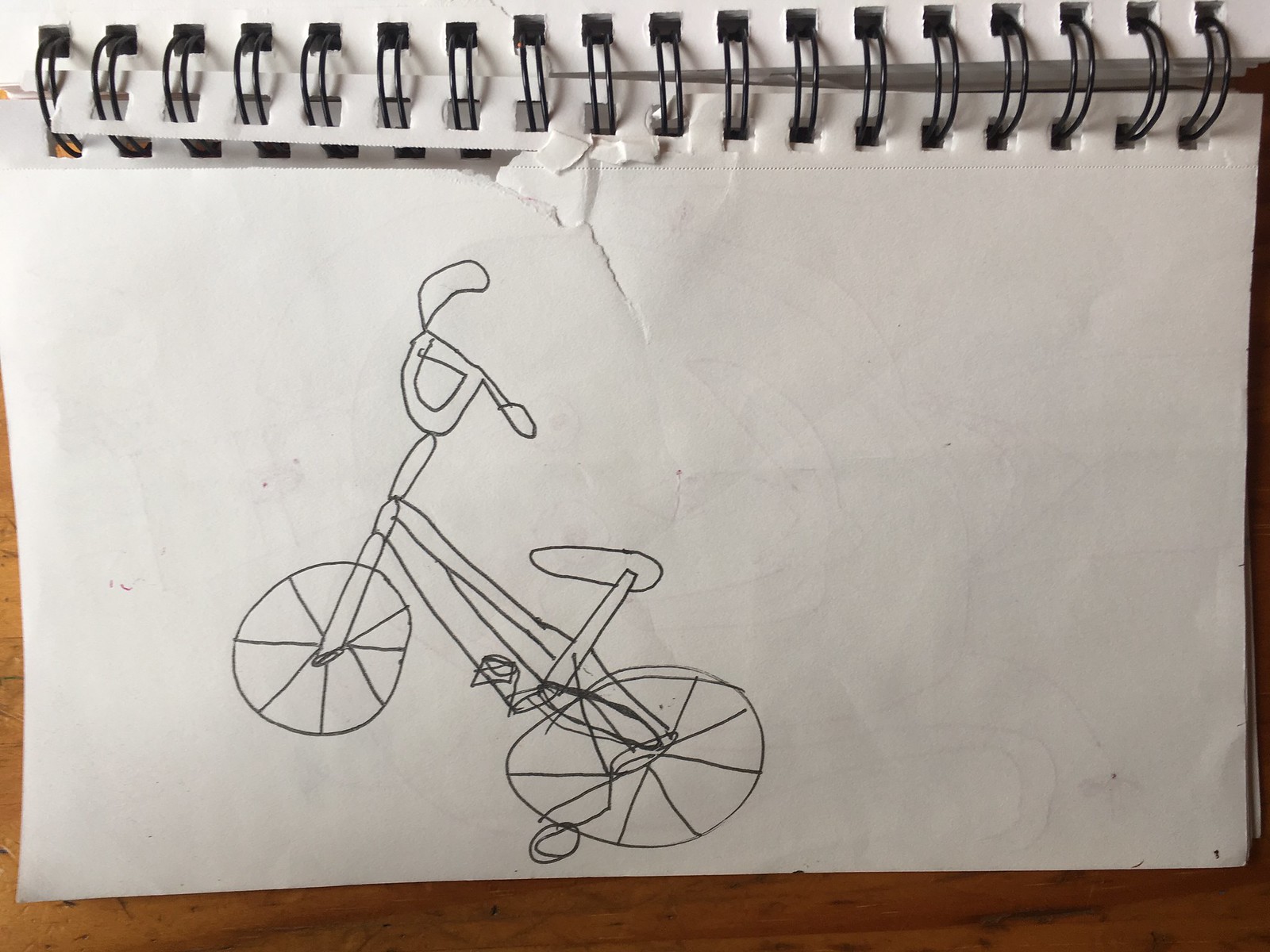This is a close-up photograph of a child's landscape-oriented drawing in a spiral-bound sketchbook lying open on a medium brown wooden table. The white piece of paper, slightly ripped near the black binder rings at the top, features an odd, pencil-drawn bicycle. The bicycle's design is simplistic and quirky, almost akin to a stick figure representation. It has two main wheels, each with seven spokes, and additional training wheels on either side. The oddly shaped bicycle includes an oblong, carrot-like seat facing left, and mismatched handlebars—one being much larger and oddly positioned compared to the other. The drawing is entirely outlined in pencil, emphasizing its childish and unrefined nature.